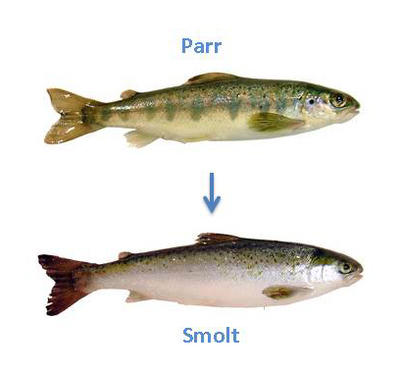This image depicts two fish set against a stark white background, arranged vertically with an arrow pointing from the fish on top to the one below. The top fish is labeled "PARR" in blue lettering, while the bottom fish is labeled "SMOLT," also in blue lettering. This suggests a developmental transition from a Parr to a Smolt.

The PARR, positioned above, features a predominantly greenish body with a yellowish-white underbelly, and its tail fin is smooth. The fish has vertical green stripes running from its dorsal to its belly and camouflaged eyes. Its upper fin on the side is notably larger compared to the SMOLT's fin.

The SMOLT below is characterized by a darker upper body with a speckled dark gray and pale pinkish-silver underbelly. Its tail fin is jagged, darker, and more reddish compared to the PARR. The SMOLT's eyes are more distinct within its color palette, standing out against its predominantly white lower body, which takes up a more significant portion of its frame compared to the PARR.

Overall, the image is a detailed representation of the transformation from PARR to SMOLT, highlighted by the clear labels and directional arrow indicating the developmental sequence.